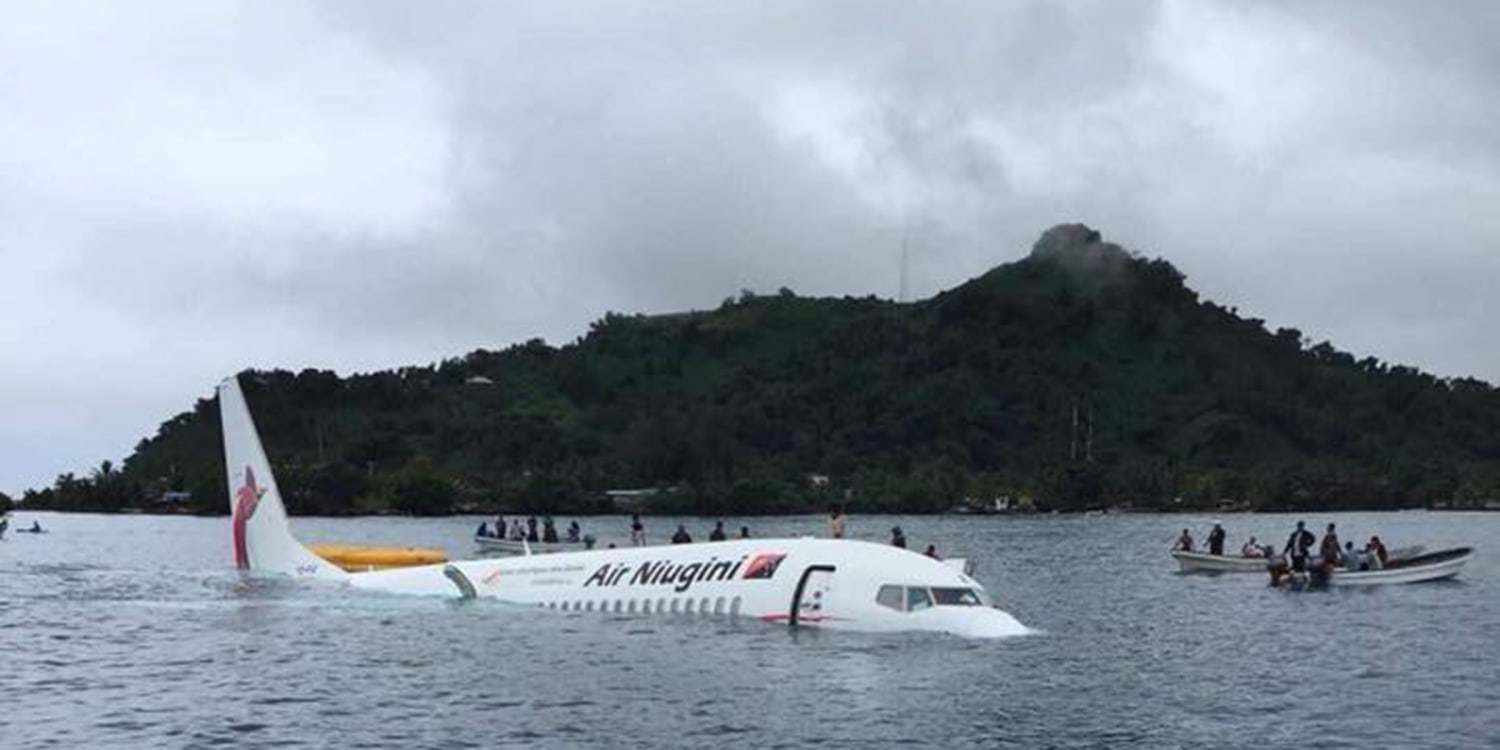In the foreground of this dramatic scene, a white Air New Genie airplane with red and blue markings appears to be sinking in a gray, cloudy body of water. Only the top half of the aircraft is visible, with the tail and parts of the fuselage sticking out above the surface. Surrounding the partially submerged airplane are several small boats filled with people, suggesting either ongoing rescue efforts or a gathering of onlookers. To the left of the airplane, a yellow raft floats, possibly indicating additional survivors or equipment. In the background, a small, densely wooded hill rises against a gloomy, overcast sky, adding to the somber atmosphere. The light blue water contrasts with the dark, cloud-covered sky, highlighting the gravity of the situation as the airplane slowly succumbs to the lake or river.